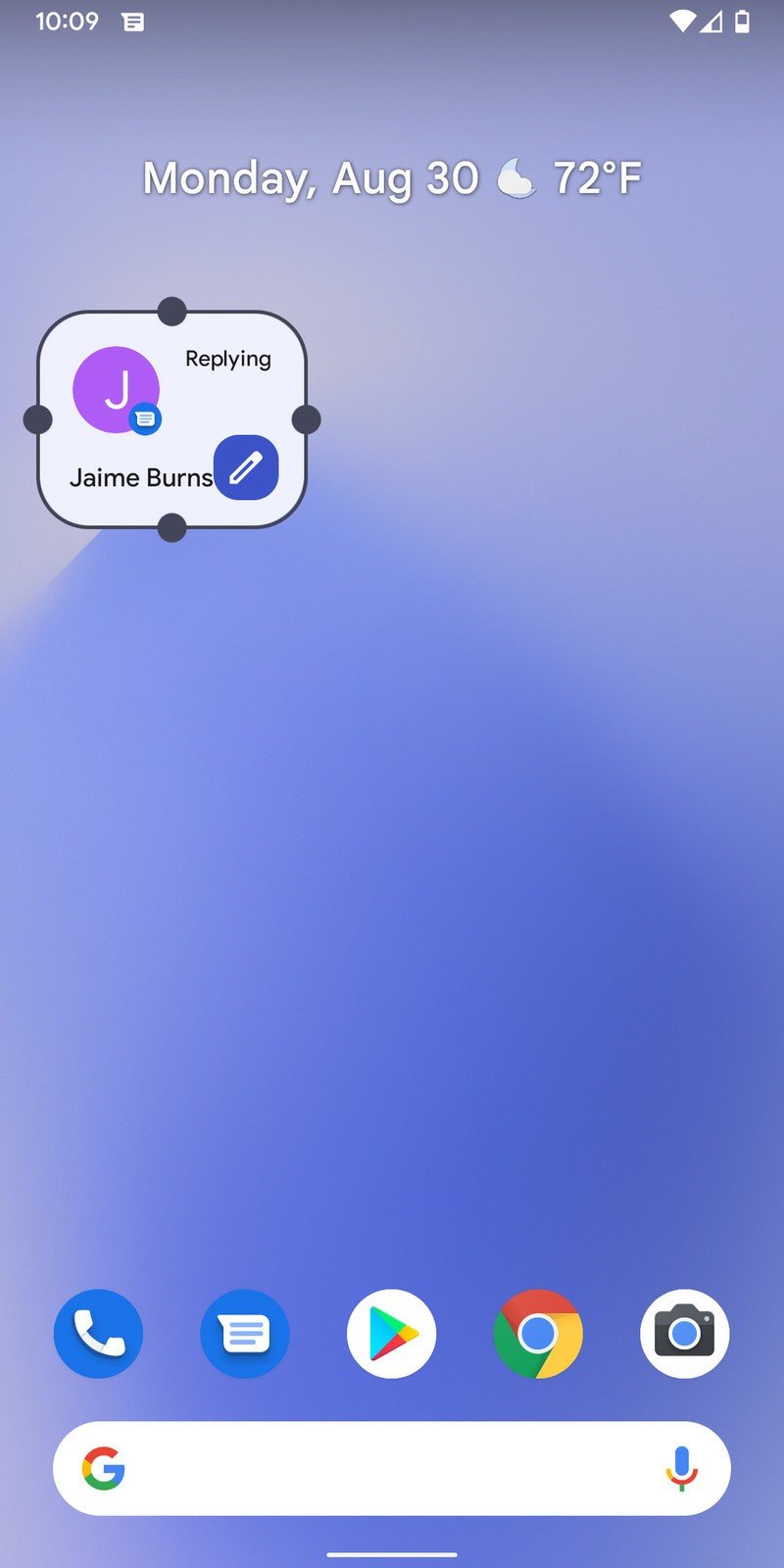The screenshot depicts a mobile device, specifically an Android smartphone. At the top of the screen, the status bar shows the current time as 10:09 AM alongside indicators for a strong Wi-Fi connection and battery level. Just below the status bar, the date is displayed as Monday, August 30th, with the temperature noted at 72 degrees Fahrenheit.

Central to the image is an open text message window that appears somewhat minimized or zoomed out, visible as a small rectangle. The background features a purple, wave-like pattern. 

Further down the screen, there are five prominent app icons situated above the home screen's navigation bar. These icons represent the Phone, Messages, Play Store, Chrome, and Camera applications.

At the very bottom, the Google search bar is displayed, characterized by a white background, a colorful Google logo on the left, and a microphone icon on the right.